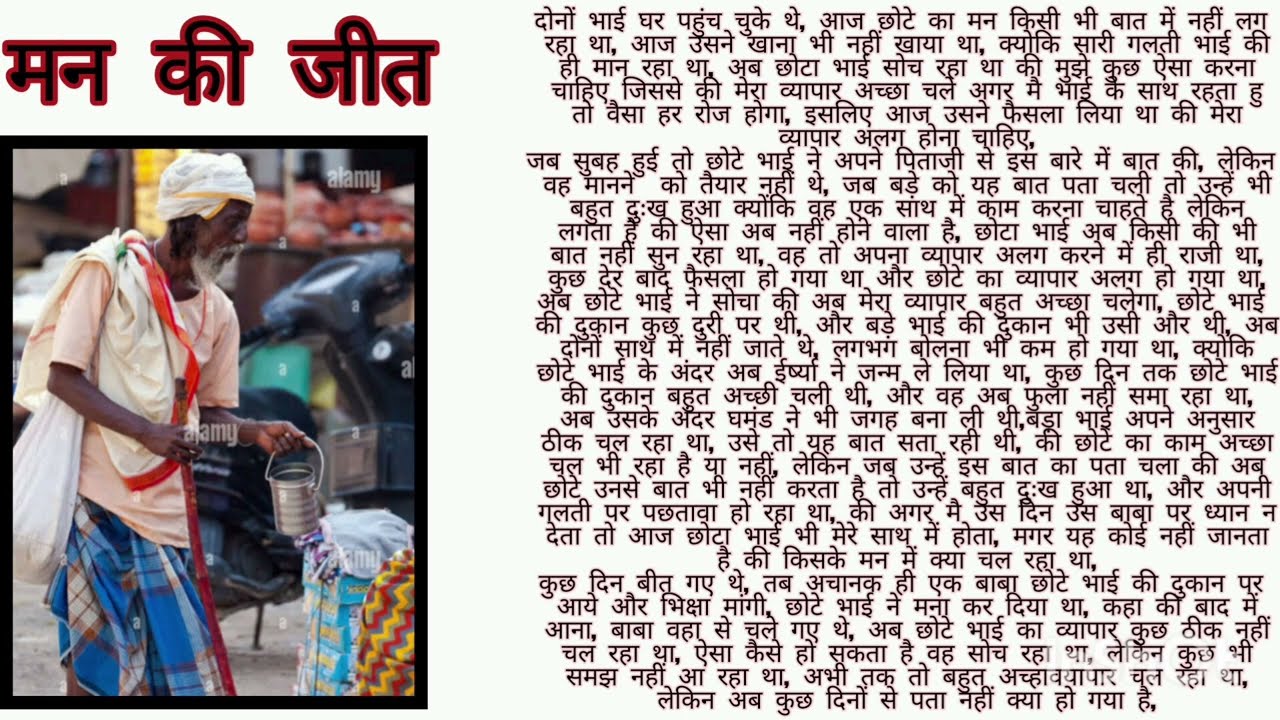The image is divided into two main sections: a large portion on the right, and a smaller, detailed inset photograph on the left. The right-hand side, taking up about two-thirds of the frame, is filled with Devanagari script, commonly used in languages such as Hindi and Marathi. This script, written in a light blue background, consists of three distinct paragraphs.

On the left side of the image, there is a striking photograph of an Indian man. Positioned below a bold title written in the same Devanagari script, the man dominates this section of the frame. He is a dark-skinned gentleman, captured in a side profile, wearing a beige-orange or pinkish t-shirt. His head is wrapped in a loose turban, and he sports a wispy gray beard and mustache. Over his right shoulder, there is a cloth draped, possibly a piece of traditional attire.

The man is dressed in a blue and brown plaid skirt-like garment around his lower body, not typical trousers. He holds a small metal pail or bucket in his right hand, while his left hand remains free. This photograph appears to have been taken in an outdoor market setting. Behind him, there is a dark-colored motor scooter, and in the background, one can discern a market stall with potential fruits or vegetables. On the lower right-hand corner of his photograph, additional items, including blue and yellow baskets, are partially visible.

The photograph features the watermark "A-L-A-M-Y" in white letters, present in the upper right corner and also above the man's left hand. The overall composition highlights both the detailed character study of the man and the extended Devanagari script, providing a culturally rich and visually engaging scene.